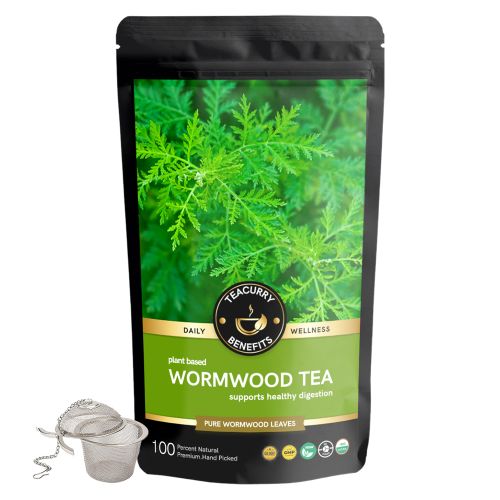This professional product image features a package of herbal tea against a white background. The packaging of the tea is predominantly black with a resealable top and a vibrant image of bright green wormwood leaves at the top. The middle section of the package highlights a circular black area where it states "Tea Curry Benefits, Daily Wellness". Below, in a light green section with white text, the packaging reads "Plant-Based Wormwood Tea Supports Healthy Digestion" and "Pure Wormwood Leaves", noting that the tea is 100% natural and premium hand-picked. To the bottom left of the package, there is a small, light gray tea sifter, or mesh diffuser, with a lid that has a silver chain attached. The sifter appears to be made of stainless steel and is roughly the size of a quarter cup, providing an elegant touch to the herbal tea set.